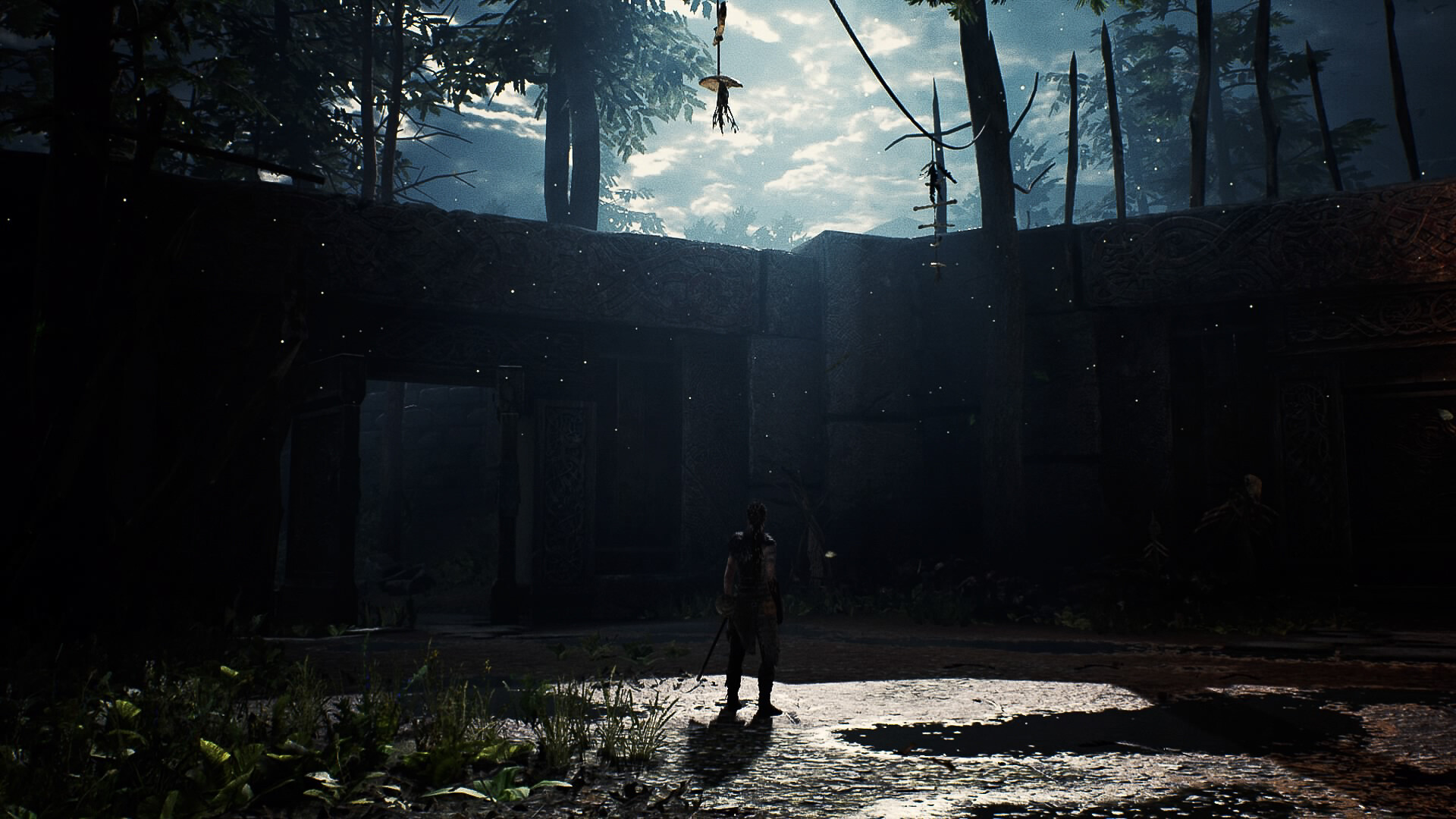The image is a widescreen snapshot from a modern video game with impressive graphics, capturing an outdoor scene under a cloudy sky where the sun struggles to pierce through, casting a diffused light over the environment. The upper part of the image, about the top 20%, is dominated by rain clouds brightened from behind by the hidden sun. Tall pine trees frame the scene on the left and right, their canopies shadowing their trunks and surrounding areas dramatically.

Central to the image, a lone character stands in a courtyard-like clearing, facing away from the viewer. The character is in shadow, giving them a silhouetted appearance that obscures finer details, though hints of leather armor and a sword suggest they are possibly geared for adventure or combat. The ground in the clearing is bare dirt with sparse vegetation, and stone walls rise around the space, lending it an air of an ancient, roofless temple or ruins.

Additionally, wooden stakes and poles with hanging wires and a suspended mini platform above the character indicate a past civilization's remnants or possibly a prepared obstacle in the game's quest. The scene is both evocative and richly detailed, placing the viewer amidst an intriguing interplay of nature, ancient structures, and impending action.